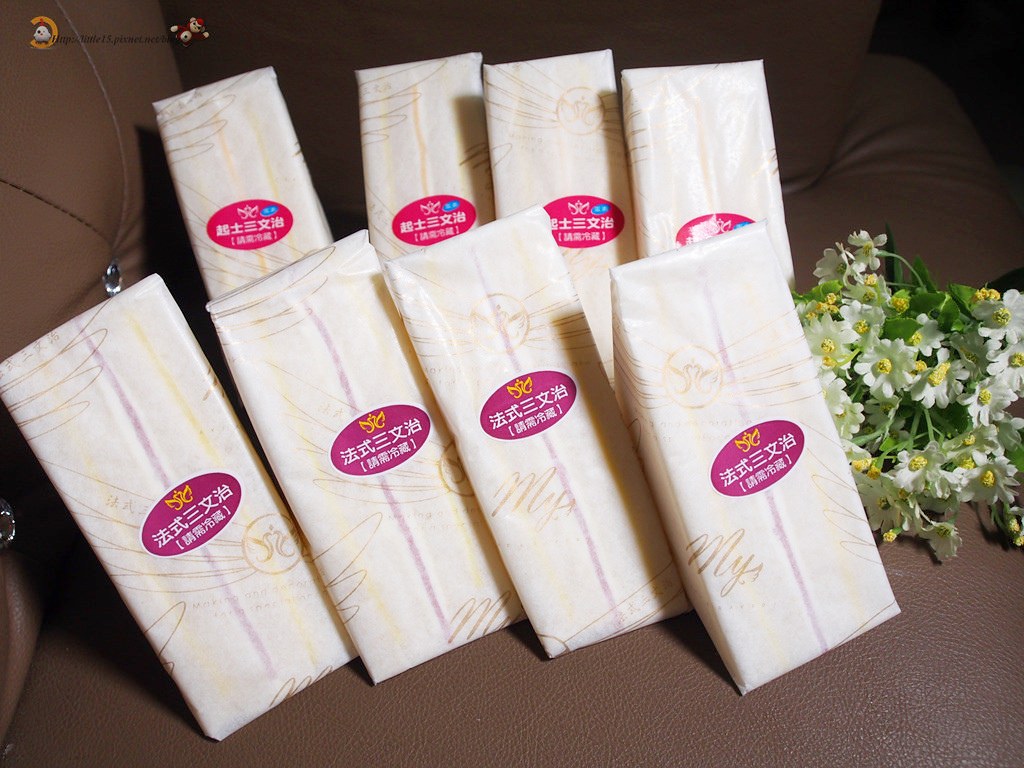The image is a color photograph depicting eight individually wrapped, triangular-shaped sandwiches placed face-on. Each sandwich is encased in a semi-translucent, off-white, greaseproof-looking paper that allows slight visibility of the sandwich's contents. The design on the paper gives a faint impression of wing-like patterns, possibly a brand logo. Each package features an elongated oval sticker at its center, bearing traditional Japanese characters; the colors of these stickers vary from pinkish-purple in the front row to reddish hues in the back row. The text, unreadable due to the Japanese script, likely includes product names or branding details, with some stickers also featuring a gold crown and others a blue item next to the crown. Through the packaging, a vertical line of pinkish and yellowish hues is visible, suggesting the cut edges of bread slices with possible fillings like butter, cheese, mayo, mustard, or even meat. The scene is set on what appears to be a brown, quilted leather chair or booth, accompanied by a cluster of decorative white flowers with yellow centers positioned to the right of the sandwiches.